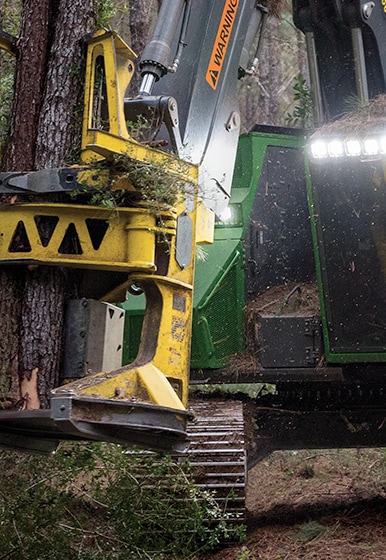The image depicts a large construction vehicle, specifically a tree-cutting and lifting machine, positioned in the middle and to the left of the frame. This machine features a crane-like arm equipped with a hydraulic grabber that reaches out to grasp trees. The vehicle has a predominantly yellow appearance with some green and black sections, and portions of it are covered in moss. Prominently displayed on its side is a warning sign, marked by a black text within an orange box and an exclamation point inside a triangle preceding the word "WARNING." The machine's base includes a tank-like tread or conveyor belt with visible black grooves. The scene is set in a dense forest with a variety of colors like greens, lighter green, gray, orange, and different shades of brown, reflecting the natural environment and the trees that surround and interact with the machinery. Additionally, there are four to five square-shaped lights on the front of the vehicle.